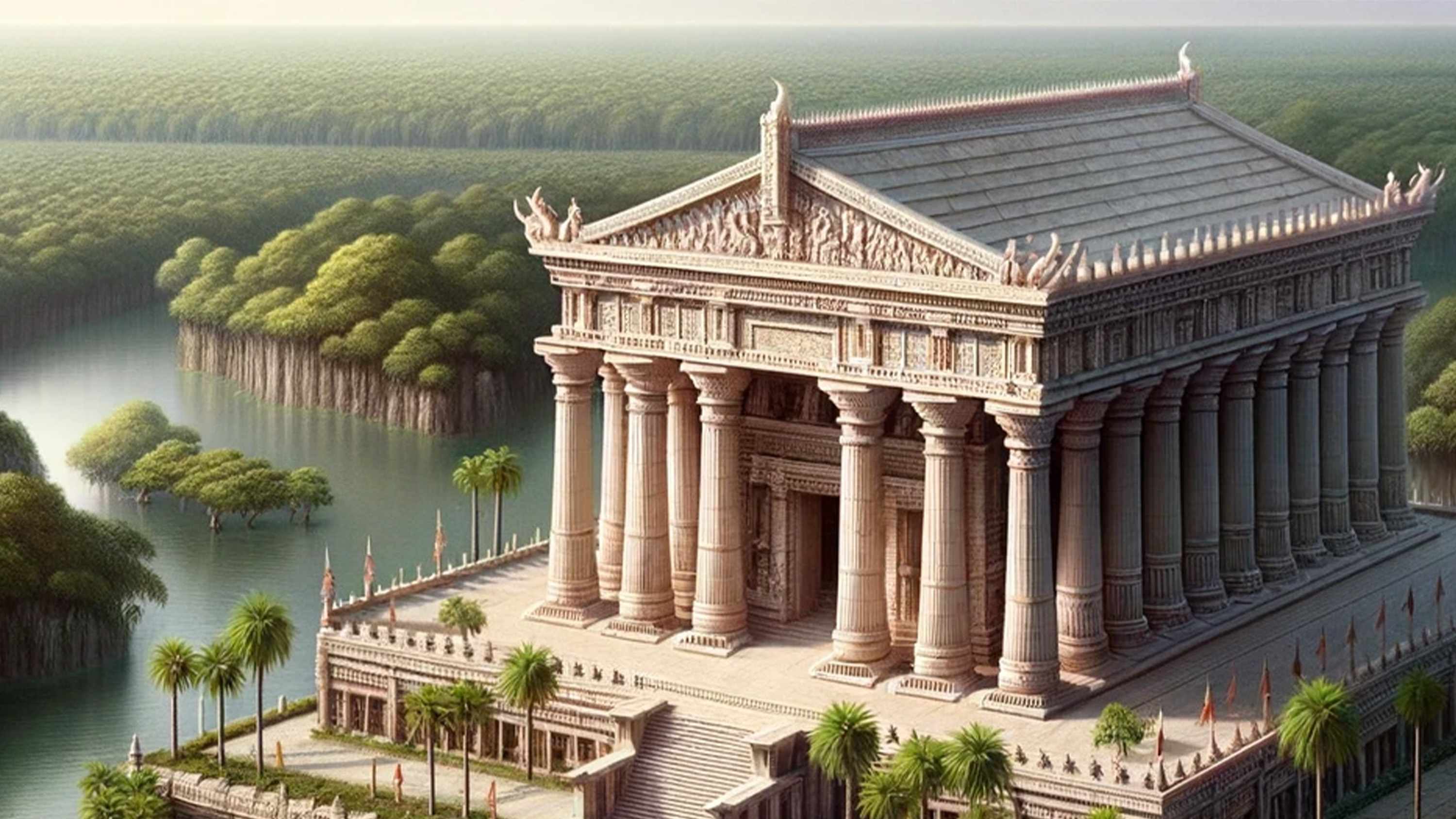This image appears to be an artistic, possibly AI-generated, rendering of a grand, ancient structure resembling a coliseum or perhaps a restored Parthenon. The building is encircled by herculean-style columns and adorned with gargoyles perched at the top, giving it a majestic and somewhat mythological appearance. It sits upon an elevated position above a vast body of water, suggesting it could be on an island or surrounded by an inlet. 

Large, steep stairs lead up to the entrance, reinforcing the building's imposing and monumental presence. The structure appears white with a faint red hue, indicating it is worn and dated. The surrounding area is lush with numerous tall palm trees, extending far into the distance, nearly obscuring the sky in places. Along one side of the structure, a series of flags add vibrant specks of color against the building's somewhat weathered facade. These multicolored flags, featuring hues of green, blue, white, and pink, offer a contrasting burst of life to the ancient edifice. The overall serene and solitary setting, without any people in sight, enhances the image's timeless and ethereal quality.